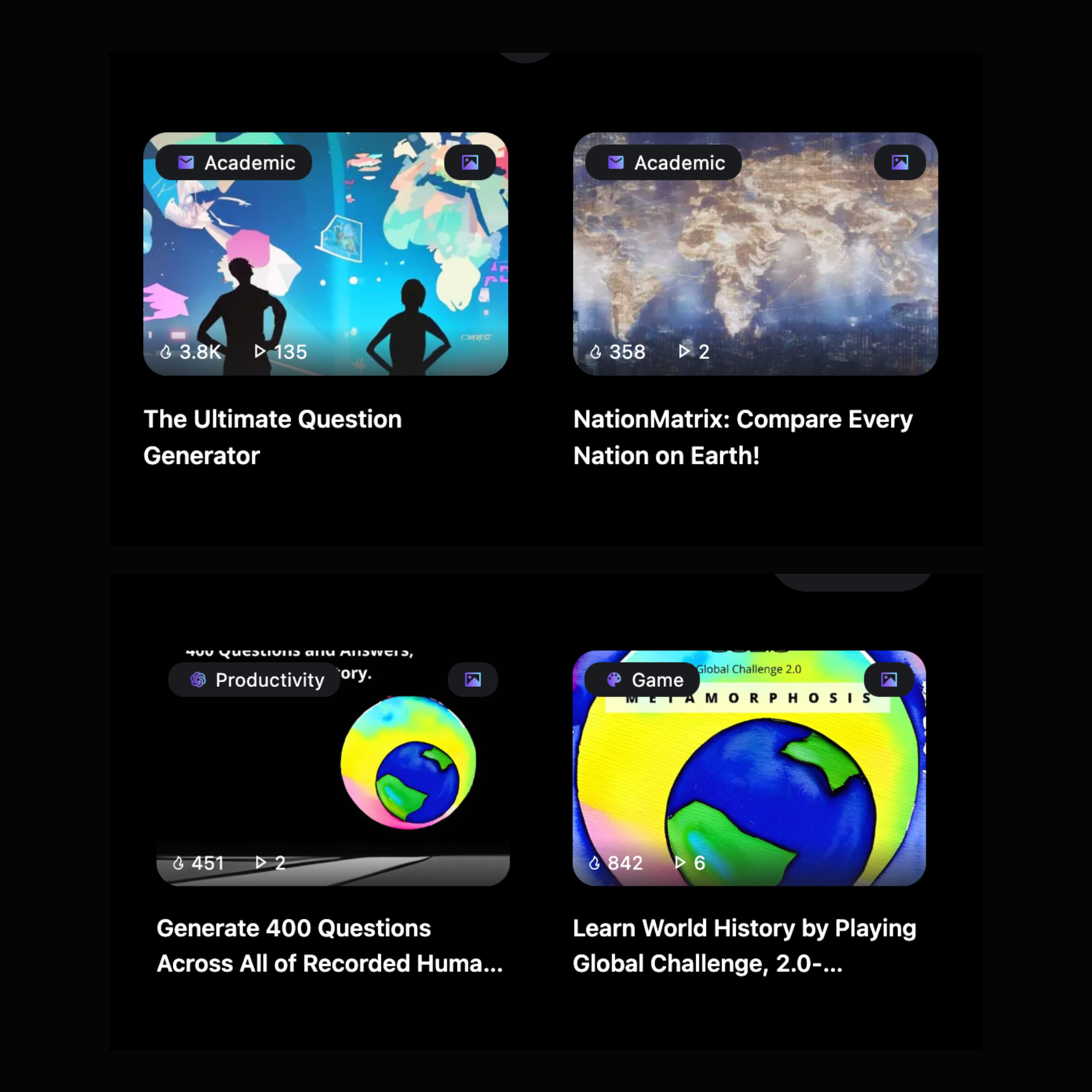This web page features a collection of educational videos, each tagged according to its subject matter. There are four videos displayed:

1. **Upper Left Video: "The Ultimate Question Generator"** - This video is tagged as academic.
2. **Upper Right Video: "Nation Matrix: Compare Every Nation on Earth"** - This brief video, potentially running for two minutes or two hours, is also academic.
3. **Bottom Left Video: "Generate 400 Questions Across All of Recorded Human History"** - Categorized under productivity, this video appears to be partially cut off.
4. **Bottom Right Video: "Learn World History by Playing Global Challenge 2.0"** - Tagged as a game, this engaging video combines education with interactive learning.

Overall, the website seems to serve as an educational hub aimed at schoolchildren or college students, offering a diverse array of subjects through visually engaging and tag-specific content.